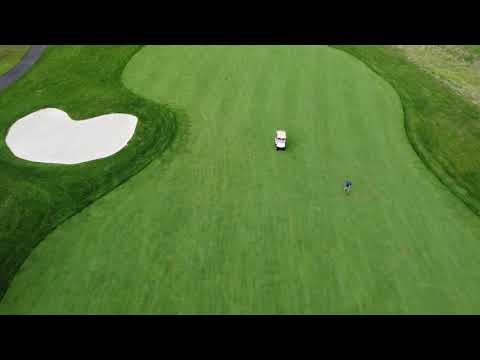This image captures an aerial view of a section of a golf course, featuring a prominent, lush green area shaped somewhat like a peanut. This central grassy area, appearing smooth and well-manicured, extends vertically from the bottom to the top of the image, tapering as it goes upwards. Positioned within this green expanse, there is a small white golf cart parked in the field, roughly 10 to 20 feet away from a man standing nearby.

Surrounding this light green section, the grass transitions into a darker, denser, taller green, indicating more natural, less-manicured growth. On the left side of the image, nestled within this darker grass, there is a white sand pit shaped like a kidney bean. This sand pit stands out distinctly against the lush surroundings. Towards the top right of the image, the ground appears rougher and less maintained, adding a wild, untamed element to the scenery.

Additionally, a sliver of a paved road is visible on the left edge of the image, marking the border between the grassy areas. This road appears to separate the main golfing area from another patch of manicured grass on the opposite side. The detailed composition of the image beautifully illustrates the varying textures and elements of the golf course landscape.